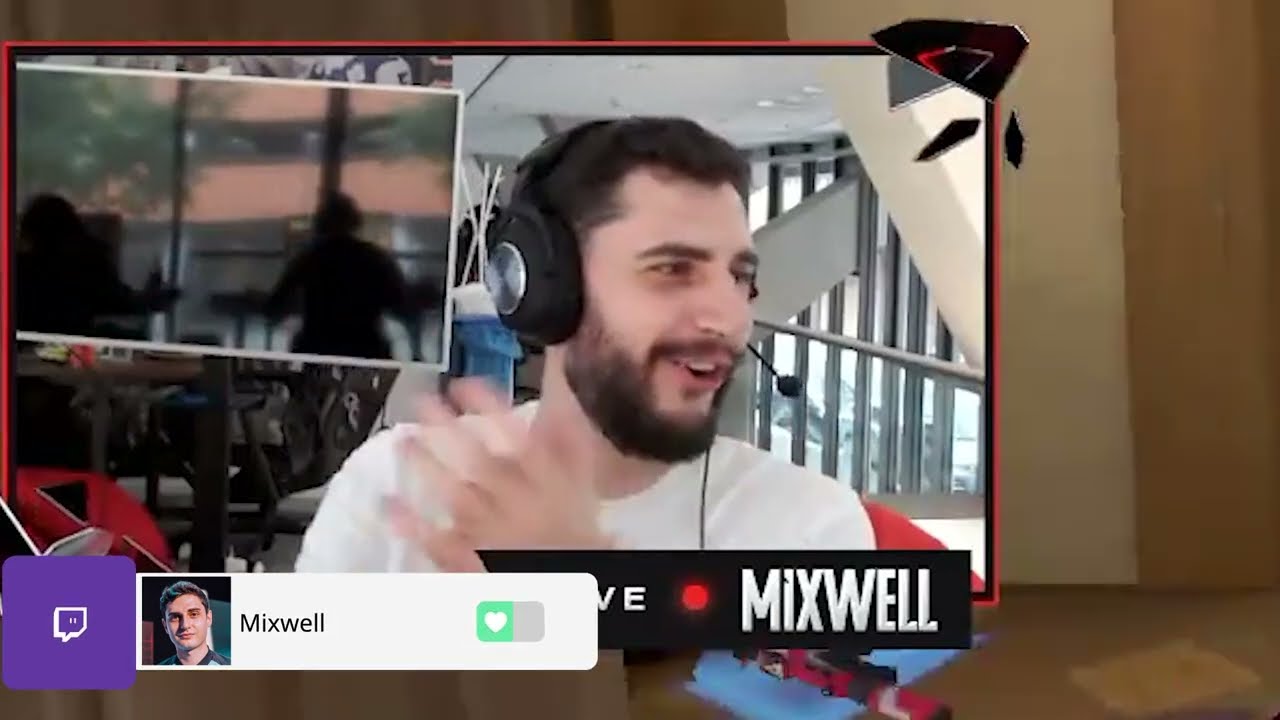The image appears to be a low-quality screenshot, likely from a live stream or a video recording. Dominating the frame is a main video feed positioned towards the upper left. It features a dark-haired man with a well-kept black beard and dark eyebrows, wearing a black headset equipped with a microphone. He is smiling, with his mouth slightly open, and appears to be in high spirits, possibly clapping his hands. He is dressed in a white shirt and seems to be seated in a red chair. Behind him, the backdrop reveals various structural elements such as thin steel railings and thicker white beams, suggesting an indoor setting that also provides a view outside.

In the lower left corner of the main image, there's a smaller inset image that displays a shadowy scene with two figures looking out a window towards what seems to be a brick building. Adjacent to this inset is a purple comment box icon with the Twitch logo, suggesting that this image might be from a Twitch stream. Just beside the icon is a white box with an avatar of a man, accompanied by the label "Mixwell," and a green heart slider icon. The text "Live" with a red dot also appears below the man's video feed, indicating that the screenshot was taken during a live broadcast.